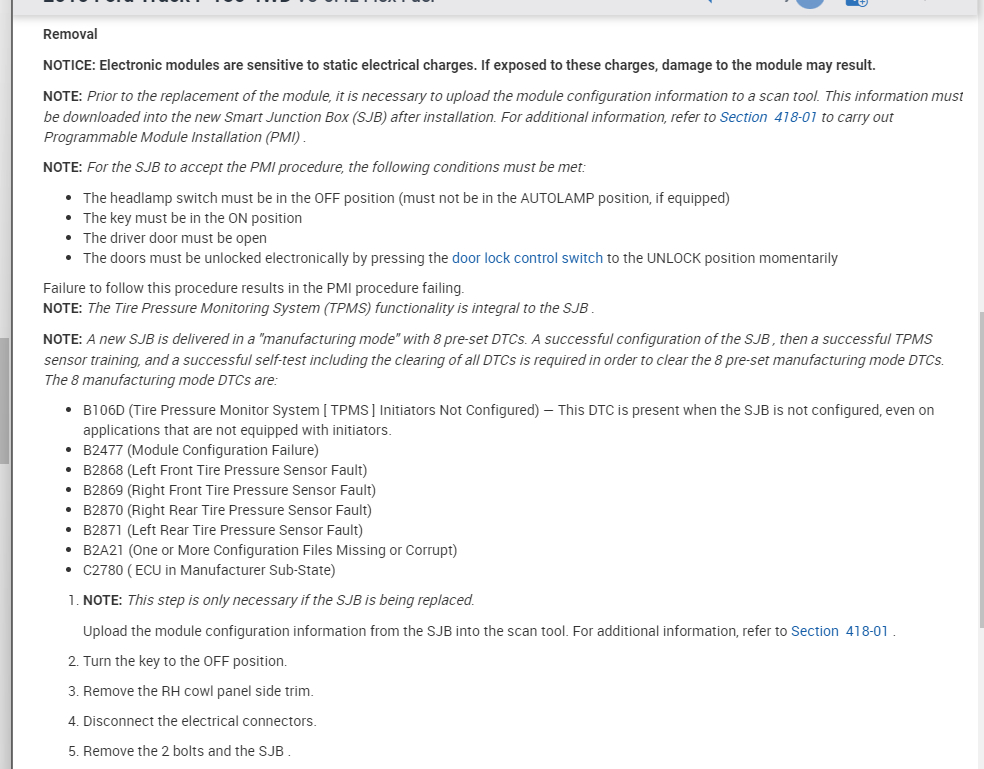This image appears to be a screenshot of a car manual page detailing instructions for handling and replacing electronic modules. The majority of the text is written in black, with certain sections highlighted in blue. The top portion of the writing is slightly cut off, but it begins with a header that includes the word "removal." This is followed by a warning that electronic modules are sensitive to static electrical charges, and exposure to these charges may result in module damage.

The manual then presents five different paragraphs, each beginning with the term "note," providing further information:

1. **First Note**: Advises that prior to the replacement of the module, the module configuration information needs to be uploaded to a scan tool. It emphasizes that this information must be downloaded into the new smart junction box after installation. For additional details, it refers to section 418-01, highlighted in blue, on carrying out programmable module installation.
   
2. **Second Note**: (Specific contents not detailed in the voice caption.)

3. **Third Note**: (Specific contents not detailed in the voice caption.)

4. **Fourth Note**: References the "door lock control switch," which is highlighted in blue. (Further details not specified in the voice caption.)

5. **Fifth Note**: Again mentions section 418-01, highlighted in blue, providing additional information relevant to the note.

The document also includes several bullet points and a numbered list ranging from 1 to 5, providing step-by-step instructions or important points.